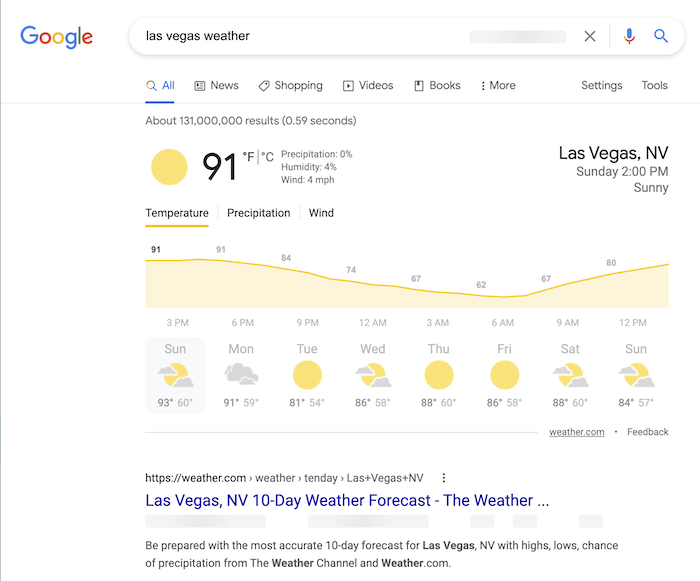Screenshot Caption: Detailed Weather Search for Las Vegas on Google

This screenshot showcases a Google search results page dedicated to the weather forecast for Las Vegas, Nevada. The familiar Google logo features prominently at the top of the page, with its distinctive coloring: the 'G' in blue, the first 'o' in red, the second 'o' in yellow, 'g' in blue, 'l' in green, and 'e' in red. Below the search bar, the query "Las Vegas weather" is clearly visible. 

Beneath the search bar, a navigation menu offers options such as "All," "News," "Shopping," "Videos," "Books," "More," "Settings," and "Tools." Currently, the "All" category is selected, as indicated by its blue text and underline.

The results display approximately 131 million entries, retrieved in an impressive 0.59 seconds. At the top of the search results, a compact weather summary is presented. A yellow sun icon indicates sunny weather with a current temperature of 91°F. Additional meteorological details include 0% precipitation, 4% humidity, and wind speeds of 4 miles per hour. The data is timestamped for Las Vegas, Nevada, at 2 p.m. on a Sunday.

Further down, the page provides a weekly weather forecast with temperature ranges for each day. Notably, the "Temperature" tab is selected, emphasized by a yellow underline. The forecast reveals the following:

- Sunday: High of 93°F, Low of 60°F
- Monday: High of 91°F, Low of 59°F
- Tuesday: High of 81°F, Low of 54°F
- Wednesday: High of 86°F, Low of 58°F
- Thursday: High of 88°F, Low of 60°F

The detailed forecast extends through the week, ending on Sunday. 

At the bottom of the screenshot, there's a clickable link to an external weather website, "hhtps.weather.com," providing a 10-day weather forecast for Las Vegas, Nevada. The link text "Las Vegas Nevada 10-day weather forecast" is highlighted in blue, ensuring easy access for further information.